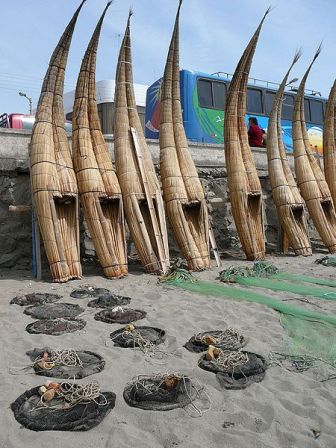In a bright blue sky setting, the image captures a beach scene dominated by homemade boats standing upright against a concrete wall. These boats, appearing to be constructed from tree bark or possibly straw and thread, feature long, pointed ends and curved hulls reminiscent of intricate fingernails. In the foreground, the tan-colored sand is scattered with small black circles containing string and rocks, while green nets are stretched out. Behind the boats, a blue and green bus with a person painted on its side adds a splash of color to the scene. A person in a red shirt is visible near the bus. Partially obscured to the left, a white building with glass windows hints at a nearby structure.